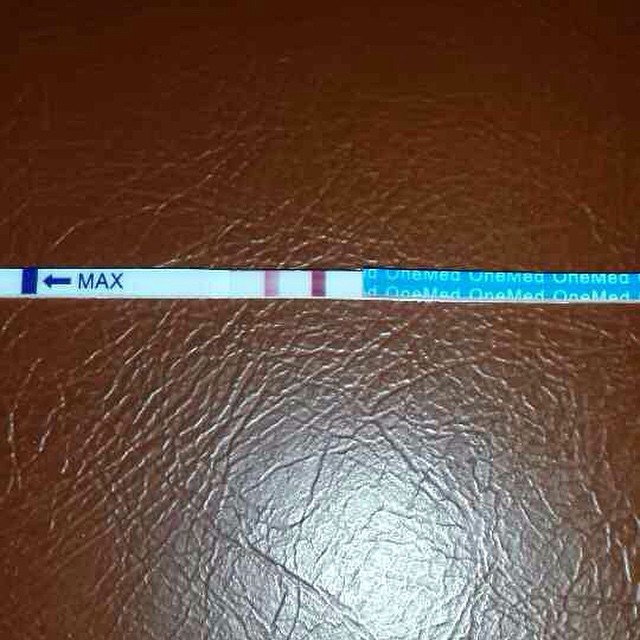The image is a close-up shot of crinkled, brown leather, showcasing its texture and rich color. The leather is shiny, with a reflection that reveals a lamp illuminating the scene. Across the middle of the photograph, there is a strap or piece of tape with repetitive text reading "One Med," and a section of the strap features a white area with the word "Max" and an arrow pointing to the right. The leather surface could be part of a leather-covered table or sofa, adding to the overall tactile and visual richness of the image. The exact purpose of the "One Med" strap remains unclear, but its presence adds an element of intrigue to the scene.